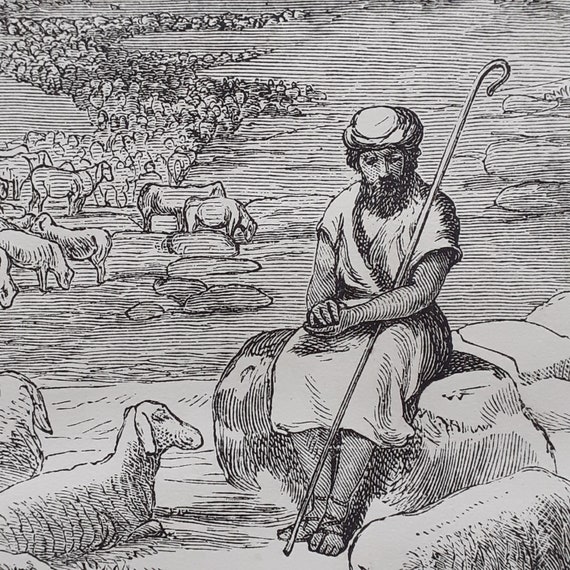In this detailed black-and-white engraving, we see a Middle Eastern shepherd taking a restful pause while tending to his flock. The young shepherd, notable for his beard and contemplative demeanor, is seated on a rock. Dressed in a calf-length white robe and a turban, he rests his shepherd's crook against his left shoulder. Surrounding him are numerous sheep and lambs, some lying close to him, while many others are dispersed in the background, grazing on the rocky mountain terrain. The flock is scattered and bunched together, meandering across the upper left side of the scene, adding depth and a sense of expanse to the composition. The engraving carefully details the rocky environment, with clusters of rocks prominent in both the bottom and top right corners, enhancing the rugged and pastoral setting. The black-and-white format accentuates the tranquil yet vigilant nature of the shepherd as he watches over his flock.